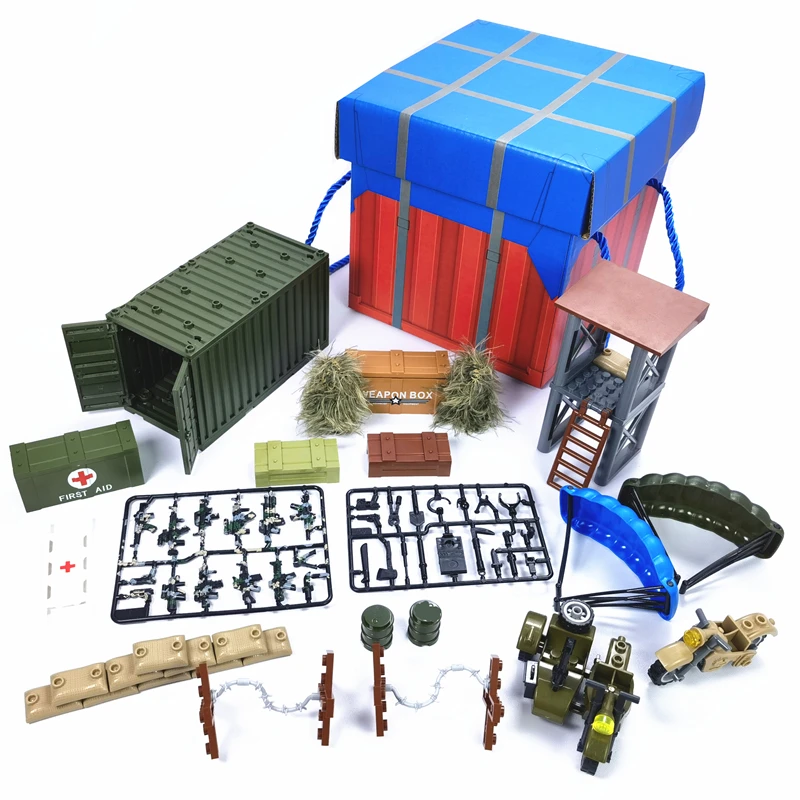The image showcases a detailed, military-themed Lego set, with various elements arranged meticulously. At the top, there is a red box featuring a blue lid with a distinct tic-tac-toe pattern. Just below and to the right, a platform and ladder lead to a Lego stand. On the left side of the image, a large, dark green shipping container constructed from Lego bricks is visible, accompanied by a green first aid kit adorned with a red cross. Scattered throughout the scene are black Lego pieces, their exact forms difficult to distinguish, but positioned near some white Lego components. A distinctive brown chain-link fence, also made of Legos, runs along the bottom. To the very right, a beige motorcycle made of Legos is situated next to two parachutes, one black and one blue. Additional items include a brown crate, various weapons in a plastic frame similar to model pieces, and a separate motorcycle with a sidecar. The assortment of pieces, some of which might be small and unconventional for a conventional toy, suggests this set may be more of an artistic statement rather than a standard children's toy, possibly commenting on the nature of military themes and exposure to violence in playthings.